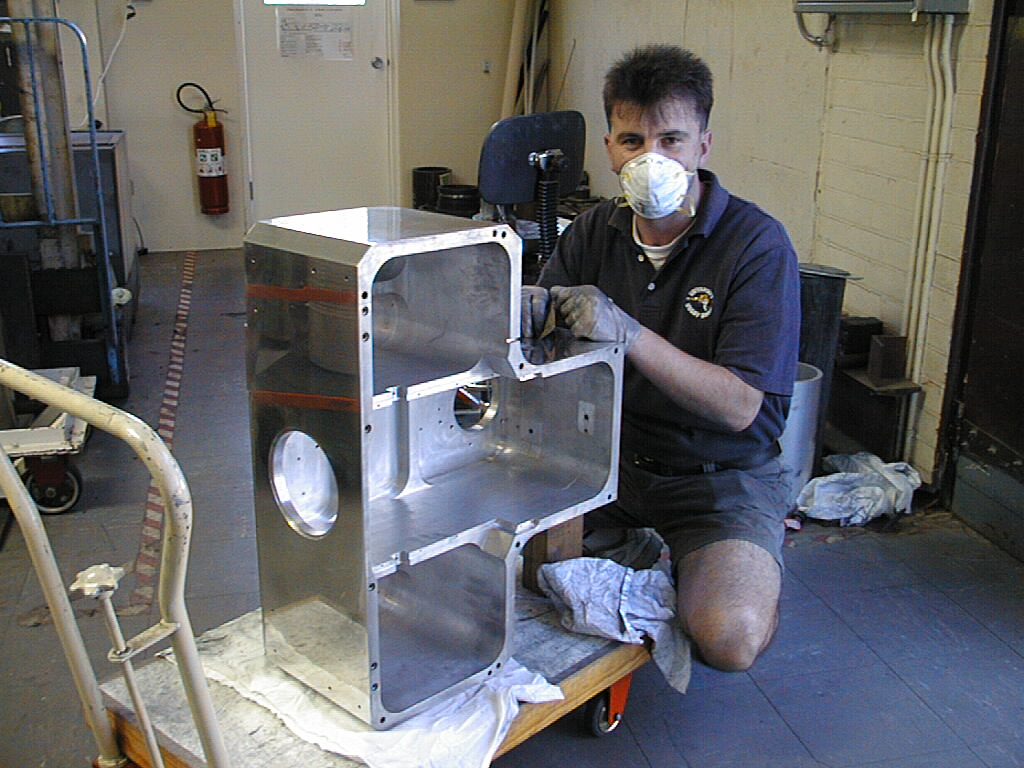This photograph captures a man in an industrial setting, possibly a factory or warehouse, kneeling beside a large, polished metal component that resembles a section of a machine. The man, equipped with an N95 respirator mask and gloves, appears to be either repairing or polishing the metallic piece. This metal object, standing on its side on a small wooden cart with maneuverable wheels, has a boxy, Tetris block-like shape with multiple chambers and various holes on its surface. Behind him, the industrial backdrop includes carts, various supplies, rags, a chair, fire extinguisher, and a door leading to another area. The man's shirt has a business logo, and he is looking directly at the camera, suggesting an interrupted moment during his work.